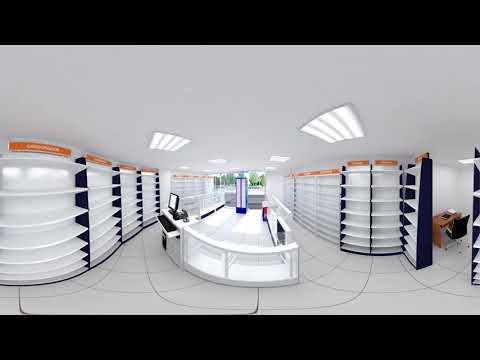This image depicts what appears to be a 3D render of a retail space, captured with a fisheye lens giving it a panoramic and slightly distorted view. The room is predominantly white, including the ceiling, which features large rectangular fluorescent lights. The floor is covered in white tiles, maintaining the overall bright and clean aesthetic. 

Along both sides of the room, there are tall shelving units with white shelves, divided by navy blue strips that run vertically. In the center of the space, a white countertop area is equipped with computer terminals and glass display cases. Notably, there's a blue display case near the door. A black keyboard can be seen on the counter, enhancing the technological aspect of the setup. 

On the right side of the image, there's a smaller room visible with a brown desk and a chair. The left side reveals an opening to the outside, where green trees are visible across the street, suggesting this space is positioned near a street or open area. The overall ambiance suggests a modern, well-organized storefront designed for retail.